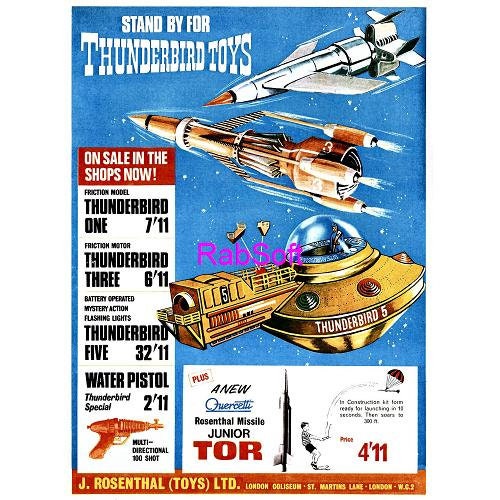The image is a vintage color advertisement for Thunderbird toys, likely from the 1970s or 1980s, set against a blue background. Prominently featured at the top is the bold text, "Standby for Thunderbird Toys." The advertisement showcases three large images of different spacecraft: a gold UFO-like flying saucer, an orangish-brown rocket ship with a red tip, and a white rocket ship. 

Adjacent text announces, "On sale in the shops now," listing various Thunderbird models such as Thunderbird 1, 3, and 5, as well as a water pistol and a missile launcher. Specific details include battery-operated mystery action flashing lights for Thunderbird 1711 and multi-directional shooting capabilities for the Rosenthal Missile Junior Tor. 

At the bottom right, there's a picture of a little boy holding a rocket, illustrated to soar up to 200-300 feet when launched and to descend with a parachute. The footer highlights the company, "J. Rosenthal Toys Limited," with additional text mentioning this business is based in London at Coliseum Street, Martins Lane.